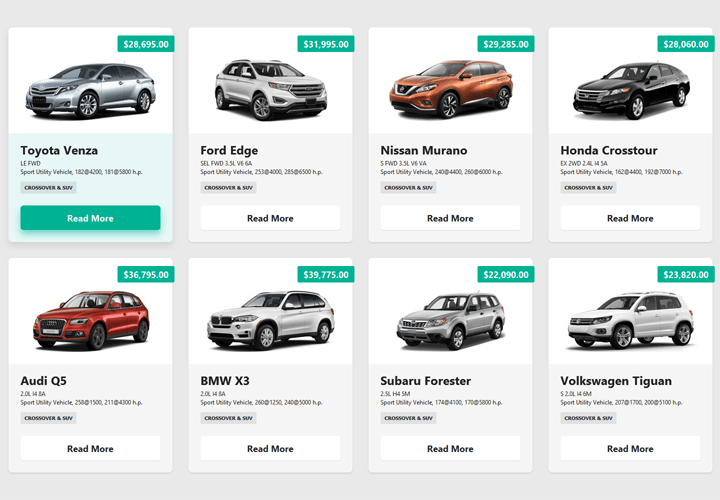The screenshot displays a neatly organized gallery of automobile listings on a gray background, arranged in two rows of four rectangular sections each. At the top of each rectangle is a white square featuring a photograph of the vehicle. Below each image, a gray section lists the vehicle's make and model in bold print, followed by additional details in smaller, black text. At the bottom of the gray section is a rectangular "Read More" button with bolded black text.

In the upper right-hand corner of each vehicle image, a green rectangle displays the vehicle's price in white text. The first car in the first row, a Toyota Venza, has been clicked, highlighting the "Read More" button in green and changing the bottom half of the section to a green background instead of gray.

The vehicle lineup in the first row features a Toyota Venza, a Ford Edge, a Nissan Murano, and a Honda Crosstour. The second row includes an Audi Q5, a BMW X3, a Subaru Forester, and a Volkswagen Tiguan.